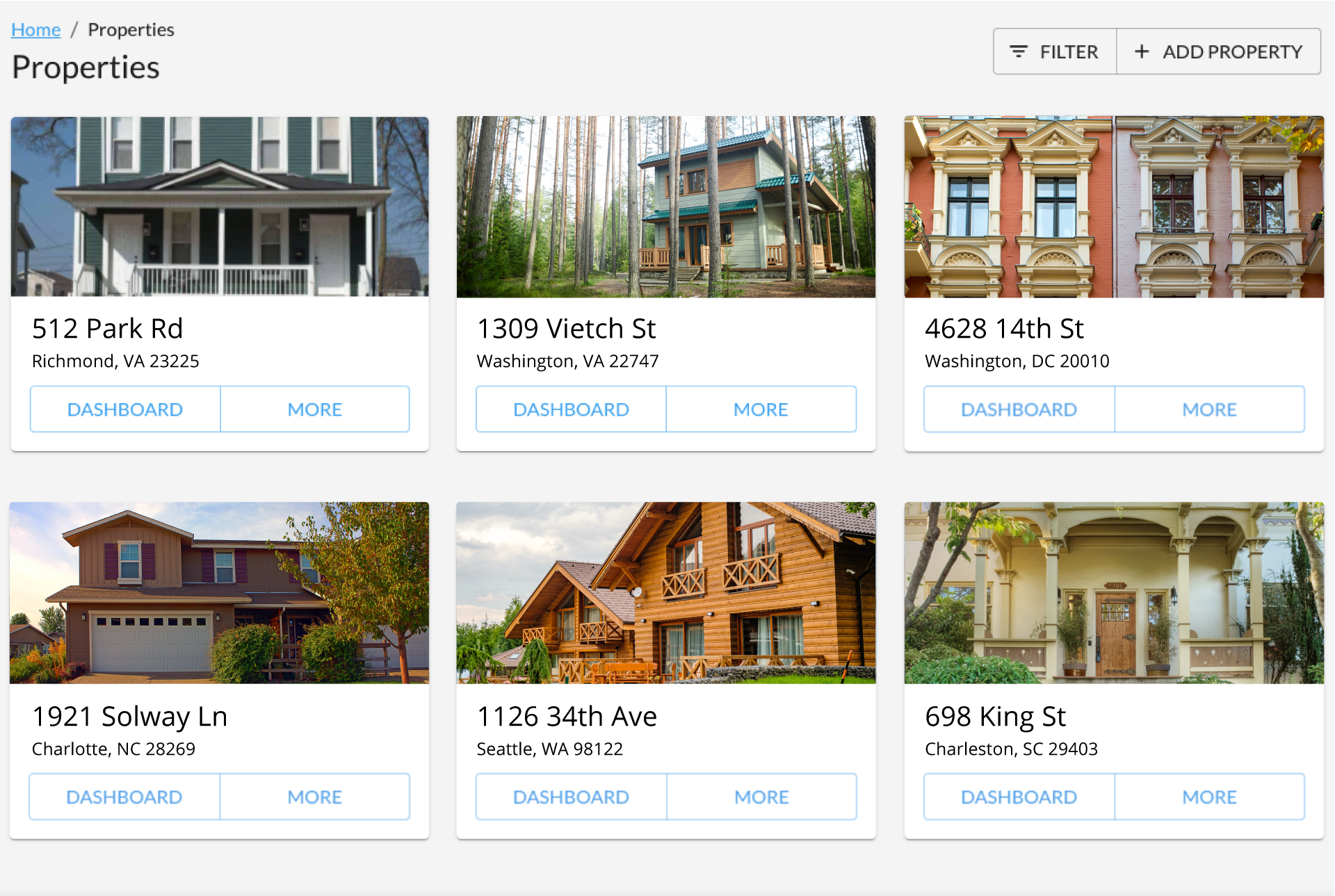The screenshot appears to be from a website dedicated to selling or renting properties. The top navigation bar features a blue header with the word "Home," followed by "Properties" in black text. In the upper right corner, two rectangular buttons are visible: one labeled "Filter" and the other with a plus sign reading "Add Property." 

The main section showcases six exterior photos of different houses, arranged in two rows of three. The first house in the upper left corner is a blue, two-story residence located at 512 Park RD, Richmond, VA 23225. Directly below each house photo, there are two buttons with a white background and light blue text, labeled "Dashboard" and "More." This structure is repeated for the remaining five houses, with each property displaying its address and the same two buttons below the respective images.